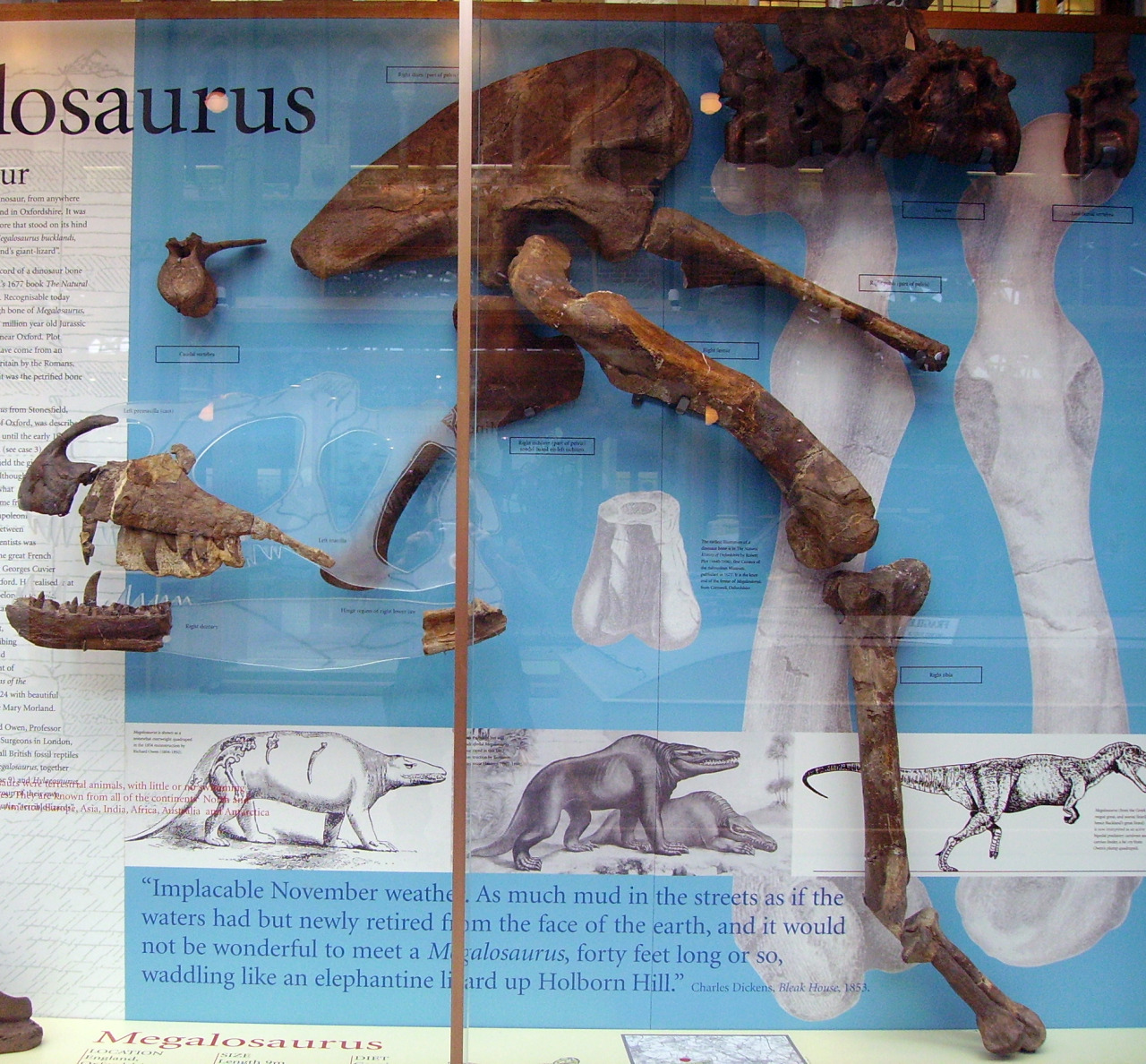This museum display features the partial skeletal remains of a dinosaur, identified as a Megalosaurus. The exhibit is set against a predominantly sky-blue background. The bones, which are brown, include portions of the skull, body, arm, thigh, lower leg, and foot. On the top left corner, partially obscured text includes the letters "L-O-S-A-U-R-U-S." Adjacent to the bones, there is an off-white or light gray strap running down the left side, which contains descriptive text about the dinosaur, although much of it is unreadable. Approximately two-thirds down this strap, there is a section displaying illustrations of three different types of dinosaurs, along with brief descriptions of each. At the bottom of the exhibit, the background returns to the sky-blue hue, displaying a paragraph excerpt that includes the phrase: "Implacable November weather, as much mud in the streets as if the waters had but newly retired from the face of the earth, and it would not be wonderful to meet a Megalosaurus, 40 feet long or so, waddling like an elephantine up Holborn Hill." This display aims to provide a detailed and evocative understanding of the Megalosaurus, both in skeletal form and within the context of historical references.